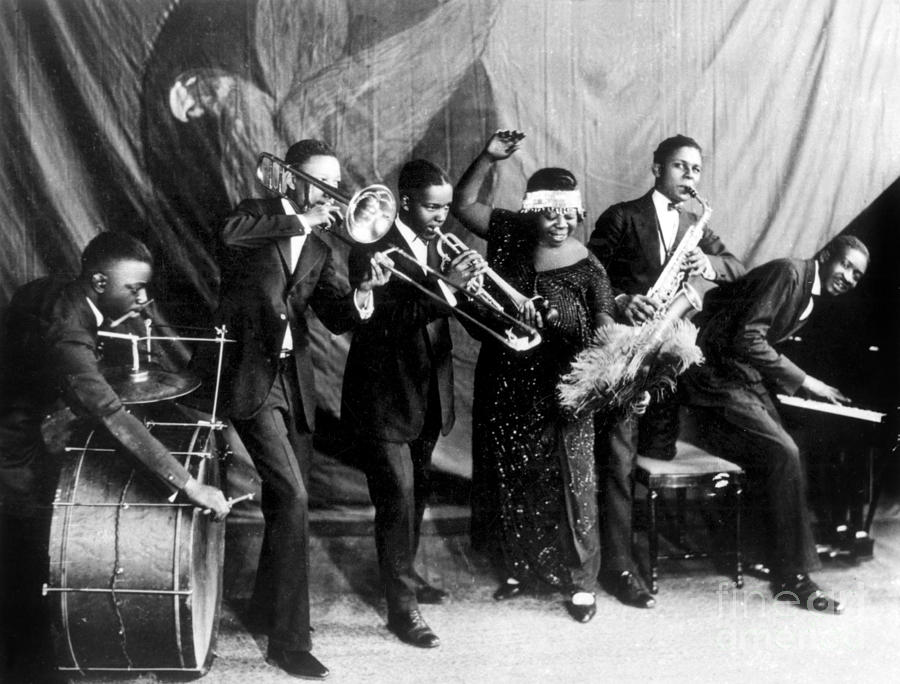This black and white photograph, reminiscent of the 1950s, captures a band of six African American musicians. The image is horizontally oriented with a faint watermark in white font, possibly saying "Fine Art America," located at the bottom right. On the left, a man is seated behind a large drum with a cymbal attached. Next to him is a musician playing a trombone with its characteristic long slide. In the center stands a woman adorned in a sequined black dress and an old-style white headband, her right hand raised as if she's singing or possibly dancing. To her left, a man plays a trumpet, while to her right, another musician handles a saxophone. The last member on the far right is positioned at a piano. All five men are dressed in formal black suits with white shirts, exuding a sense of joy. The background features a hanging cloth, possibly a stage curtain, with a hint of a banner displaying an indistinct bird design. The pristine white floor beneath them adds to the photograph's vintage charm.